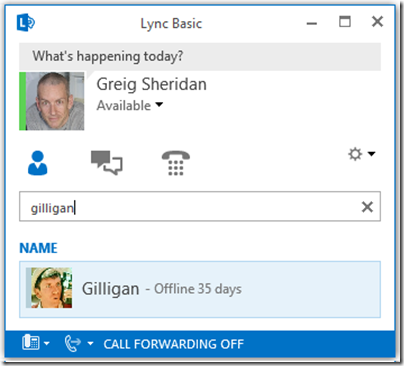Here is a cleaned-up and detailed caption for the image:

"In this screenshot from a contact application, the top center of the window displays the text 'Link Basic.' In the upper right corner, there are icons for minimizing, resizing, and closing the window. A chat bubble with the message 'What's happening today?' is shown emanating from a profile picture of a man named Greg Sheridan, whose status is marked as 'unavailable.'

A search bar has the text 'Gilligan' entered in it. Below this, the application displays search results under the heading 'Name.' The result includes a profile icon of a man looking off to the right, showing the name 'Gilligan' with a status of 'Offline for 35 days.'

At the very bottom of the window, there is a phone icon followed by the text 'Call Forwarding Off' displayed in white font."